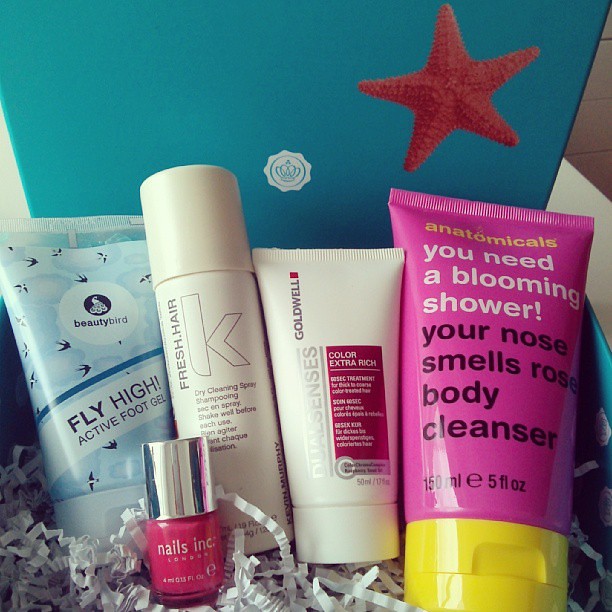This image depicts a well-arranged beauty gift box, likely intended as a thoughtful present or a curated collection of personal care items. The central focus is on an array of five different products, all neatly nestled within protective packaging designed to prevent damage during transit. The box itself has an aqua blue background, adorned with a white crown logo and a red starfish on the right side. 

In the center of the photo, from left to right, are the following items:
1. A tube of Beauty Bird Fly High Active Foot Gel, featuring a blue design with bird imagery.
2. A bottle of Nails Inc. nail polish in pink, with a distinctive silver cap.
3. A cylindrical container of Fresh Hair Dry Cleaning Spray by K, characterized by its off-white color and detailed text including product instructions.
4. A white 50 ml bottle of Goldwell Dual Senses Color Extra Rich Treatment, specifically formulated for thick to coarse colored hair, embellished with red and other colored logos.
5. A pink 150 ml bottle of Anatomicals You Need a Blooming Shower, Your Nose Smells Rose Body Cleanser, which stands out with its lemon-green cap.

The scene appears to be captured indoors, potentially either in someone's home or in a store that specializes in beauty products, with lighting suggesting it is midday. The color palette spans a range from classic pinks and reds to soothing blues and neutral whites, enhancing the visual appeal of the gift box.